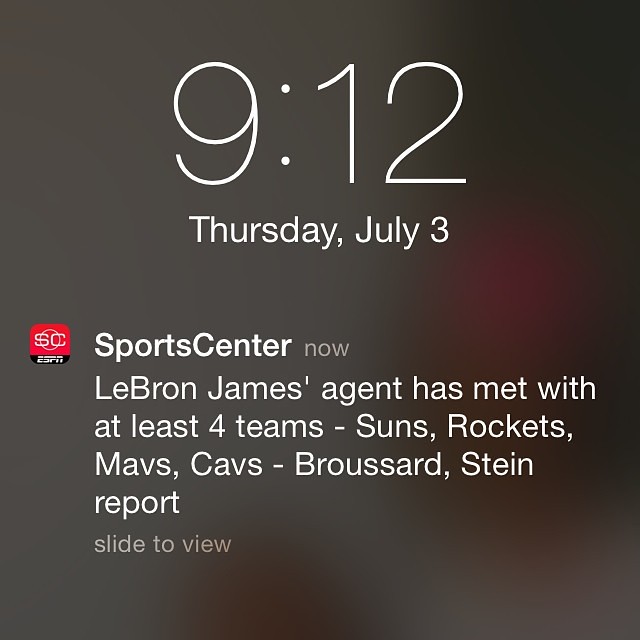This image captures a square-shaped notification from ESPN displayed on a phone screen. The background is a steel gray color, accentuated by subtle lighted areas along the right side midline. There are blurry red spots with yellowish-green outlines, one near the bottom left of center and another more diffused spot elsewhere. At the top of the square notification, in large white letters, it indicates the time as "9:12" followed by "Thursday July 3rd" in smaller, bold white text. Below this, to the left, is a red square with a black footer; the black footer contains the text "ESPN" in white. Inside the red square, there is a white circle featuring the letters "S" and "C" intertwined. Adjacent to this, the words "SportsCenter" are prominently displayed in bold white text, followed by "Now" in gray. Beneath this, white text relays the headline: "LeBron James' agent has met with at least four teams - Suns, Rockets, Mavs, Cavs - Broussard, Stein report." At the bottom of the notification, instructions in gray state "Slide to view."